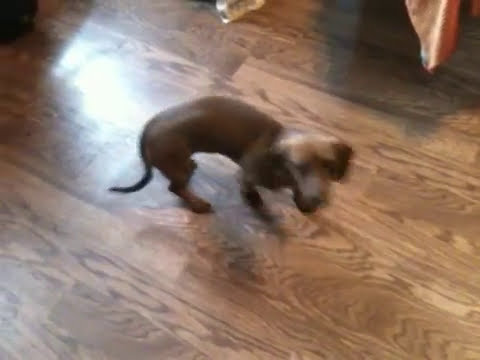The image is a slightly blurry, overhead shot of a small, brown dog, possibly a dachshund or beagle, standing on a light brown, glossy wooden floor. The dog, with its big ears and short tail curved upwards, is in motion, arching its back slightly and lifting one of its front legs as if running or barking. Light is shining down on the floor, creating reflections, while the top right corner of the image features some kind of fabric or clothing draped over chairs. There's a shadow beneath it adding to the scene's dynamic feel. The dog appears to be looking upwards, seemingly at the camera, with an expression that could be interpreted as curious or concerned.